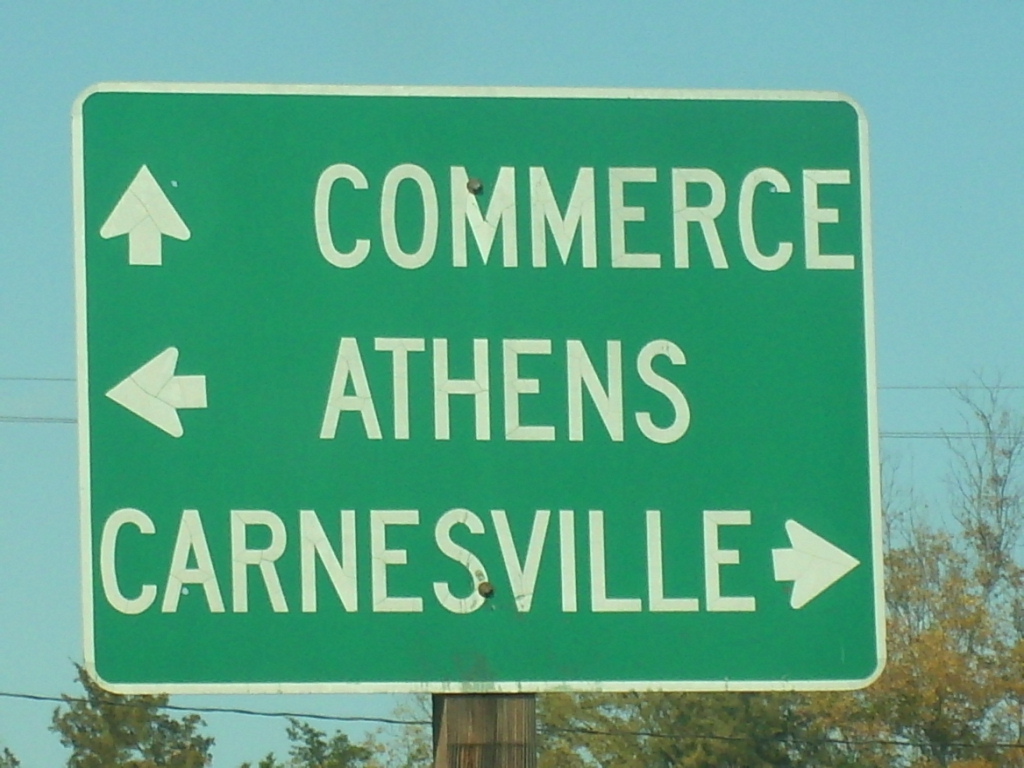The image showcases a close-up view of a large, green highway sign, affixed to a sturdy wooden post. The sign prominently displays three place names—Commerce, Athens, and Carnesville—each accompanied by directional arrows: an arrow pointing straight ahead for Commerce, an arrow pointing left for Athens, and an arrow pointing right for Carnesville. The white reflective perimeter and lettering make the sign easily visible, even in low light. The scene is set during the daytime, under a sky that is a grayish-blue hue. In the background, mature trees, including some with orange leaves and some evergreens, are visible, along with power and telephone wires running across the sky. The primary focus of the image is the road sign, with its idyllic, nature-filled background adding depth and context.